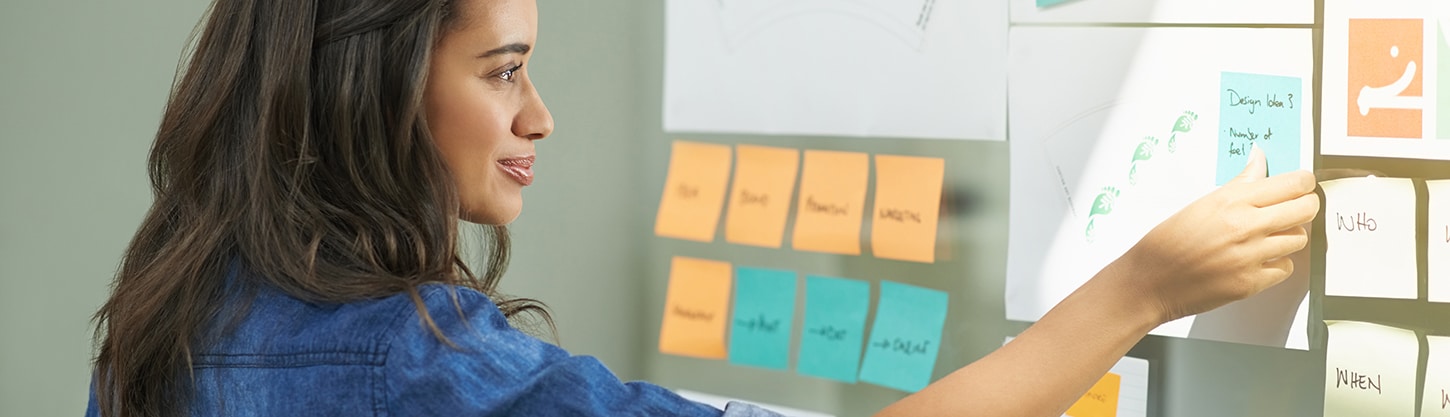In this horizontally oriented photograph, a woman with long, dark brown hair and tan skin is shown in side profile, slightly smiling as she reaches up to place a green post-it note on a large white piece of paper attached to what seems to be a glass room divider. She is wearing a denim top with the sleeves rolled up and is looking intently at the note, which appears to say "design something." Surrounding her are various other sticky notes: a row of orange and cyan ones to her left, and several light yellow notes to the right with words like "who" and "when" written on them. The white paper features green patterns resembling footprints, adding an extra layer of detail to the scene. The background of the photograph is a dark white color, suggesting an office or school environment.